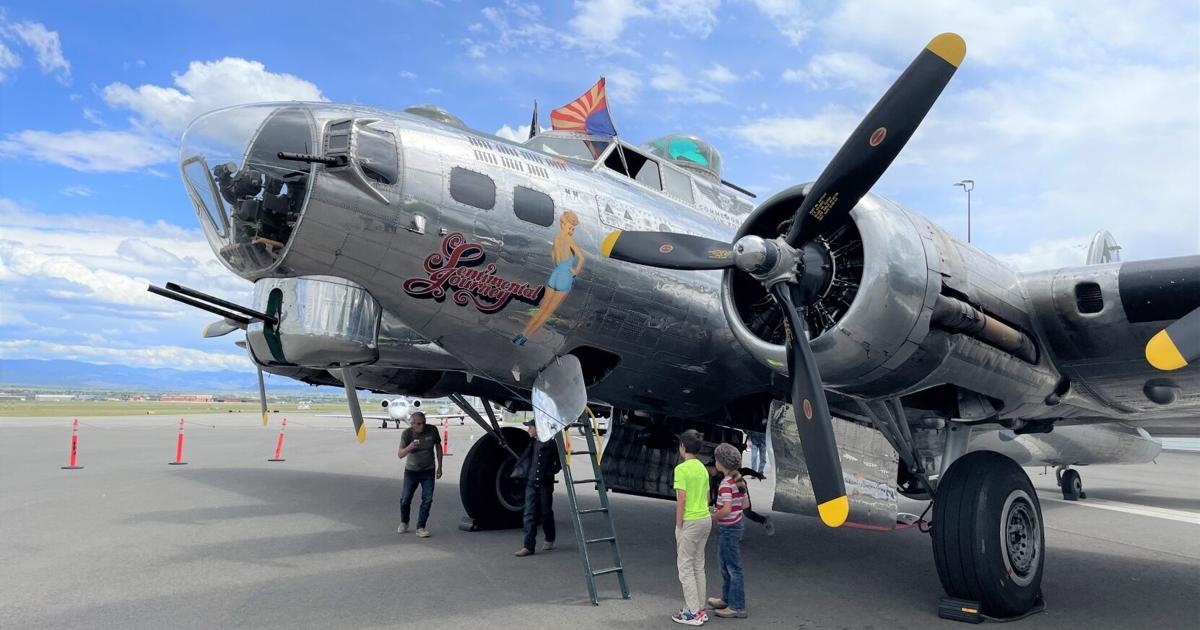The image depicts a vintage, silver World War II-era bomber plane named "Sentimental Journey," as indicated by the prominent red script on its side. The aircraft has a striking stainless steel appearance with highly polished metal and black propellers featuring yellow tips. An illustration of Betty Grable in her iconic swimsuit pose, turning to look at the camera, is painted next to the text on the plane. The scene includes a small green ladder leading up to an open hatch beneath the plane, with four people visible nearby: two male adults, one wearing a bright yellow shirt and another in a red and tan striped shirt, along with a child dressed in black and another child in a gray shirt and jeans holding a coffee cup. Additionally, a flag with red, white, and blue colors is mounted at the top of the plane, though it does not resemble the American flag. In the backdrop, a second plane is partly visible, indicating an airfield setting.